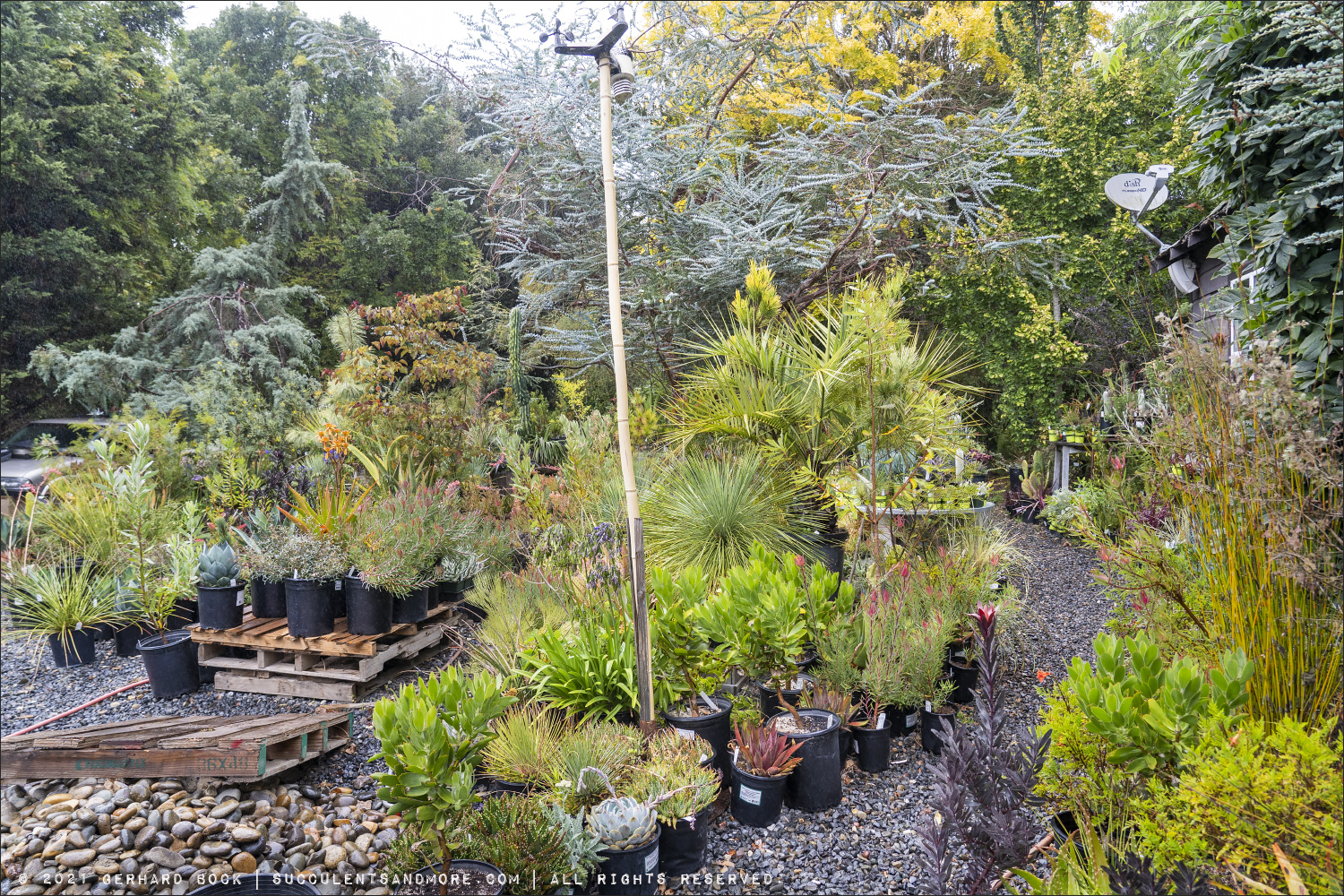The image captures a picturesque garden brimming with an array of trees, bushes, and vibrant flowers. A gravel pathway winds from the right, curves to the front, and extends along the foreground. On the left side and foreground, there are numerous black plastic pots filled with flowers, with some of these pots arranged on a wooden pallet. A tall pole stands prominently in the middle of the image, topped with what appears to be a triangular structure likely functioning as a sprinkler. In the background, large, mature trees, potentially including pines, form a lush backdrop. Additionally, a satellite dish can be seen on the right side of the image, and some faint white text is present at the bottom left. The sky above is overcast, contributing to the serene ambiance of the garden scene.